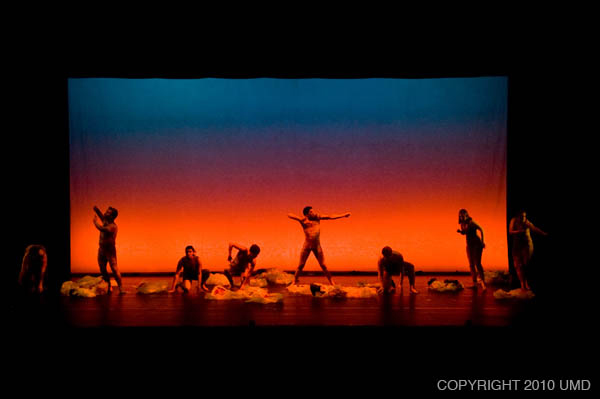This photograph captures a dramatic scene from a play or musical featuring several performers on stage. The backdrop of the stage resembles a vibrant horizon, transitioning from a deep blue at the top, through purple, to a fiery orange-red at the bottom, evoking a sunset or sunrise. The central figure, a man who appears to be unclothed, stands poised in a stance as if drawing back a bow. Surrounding him are other performers—both men and women—depicted as cavemen, engaged in dynamic movements that suggest stabbing the ground and crouching. Scattered across the stage are props that resemble sleeping bags or bedding, adding to the primal and raw atmosphere of the scene. The overall tableaux suggest a primitive and intense moment within the context of the play.